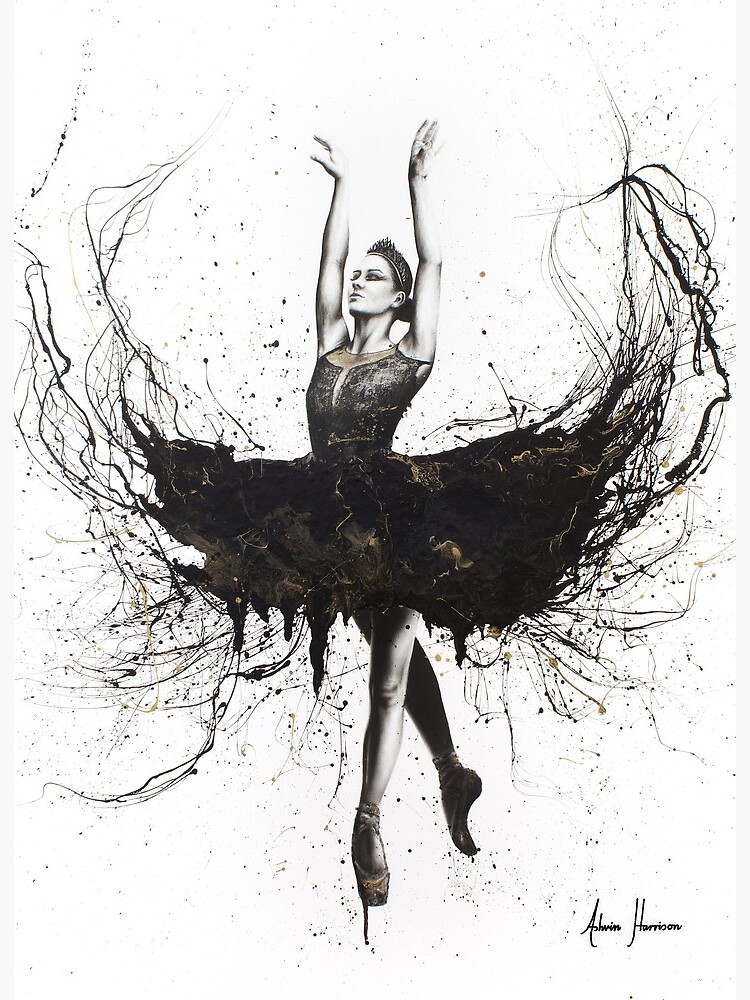This black-and-white illustration of a ballerina captures her in a graceful pirouette pose. With her arms elegantly raised overhead, she wears a regal black tiara and winged black eyeliner that accentuate her poised expression. Her black leotard, made from a lacy material with a front slit, complements her thick, flowing tutu adorned with gold accents. The tutu fans out dramatically, creating an almost inkblot-like effect with lines and dots extending in all directions, giving the impression of motion and air lifting the fabric. Standing on pointe, her right ballet shoe has a paint drip extending downwards, adding to the artistic flair of the piece. Set against a white background, the detailed shading and intricate line work enhance the surreal beauty of the scene. The rectangular image, taller than it is wide, is signed by the artist in the bottom right corner, which appears to read "A. Harrison."